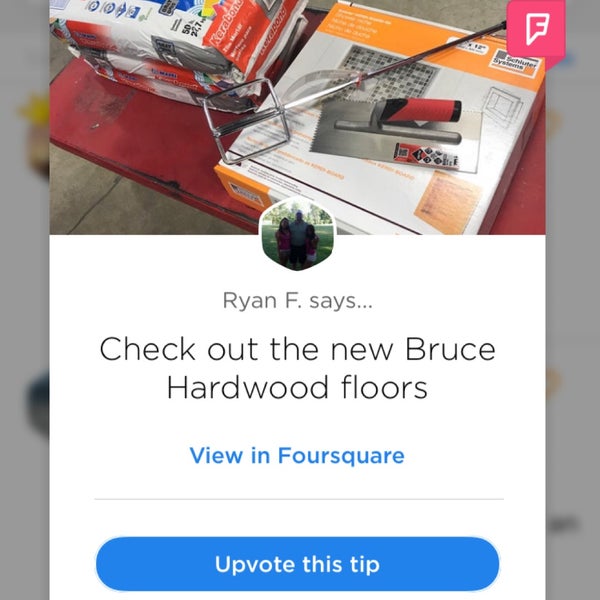In the background on the top left, there are several bags. On the top right, there is a metallic object that resembles a sword handle, but is likely a tool for a specific purpose. There's also a noticeable red square with the letter "F" in it. An orange box depicts something akin to bathroom tiles. Additionally, there's a metal tool with a handle, seemingly used for flattening out materials. In the foreground, a person stands with their family on a grass-covered area. A caption by Ryan F reads, "Check out the new Bruce Harwood Forest view on Foursquare." Above this caption, within a blue rounded circle, the phrase repeats, emphasizing different kinds of text presentation.